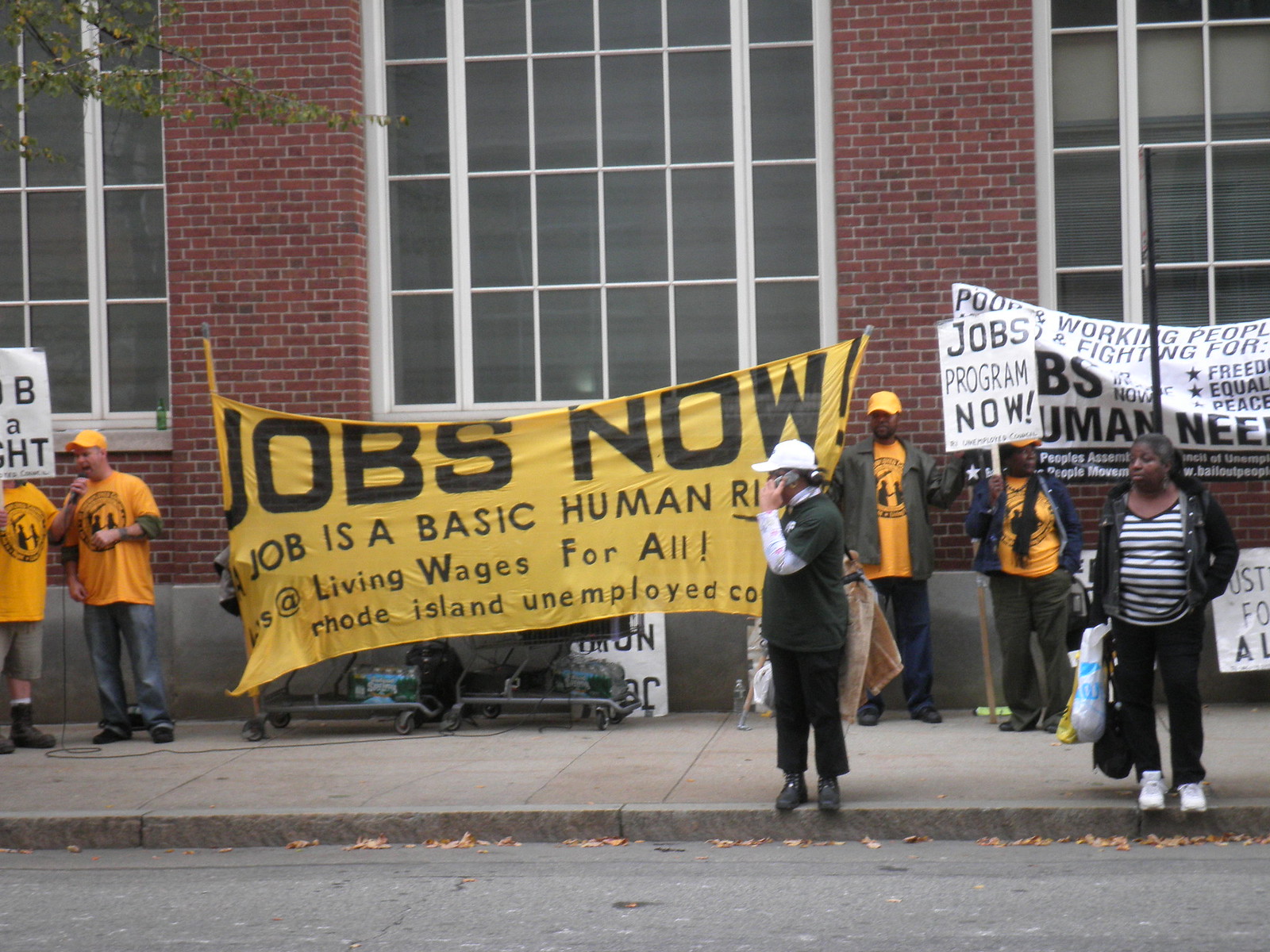In front of a large brown brick building with three massive white-framed windows, a group of people has gathered on the sidewalk, seemingly in protest. The most prominent banner, a bright yellow one that reads "A job is a basic human right at living wages for all, Rhode Island unemployed," is held up by one person and secured in a shopping cart that also contains bottled water, indicating their prolonged presence. Many in the group wear matching yellow T-shirts adorned with a circular logo featuring people inside, and they hold signs with slogans like "Jobs Program Now" and "Jobs Now." Among them, a person wearing a white cap stands on the curb, engrossed in their cell phone. There are also other individuals on the scene in regular clothing—black, white, and striped shirts—some carrying shopping bags or using their phones, who appear to be bystanders rather than part of the protest.